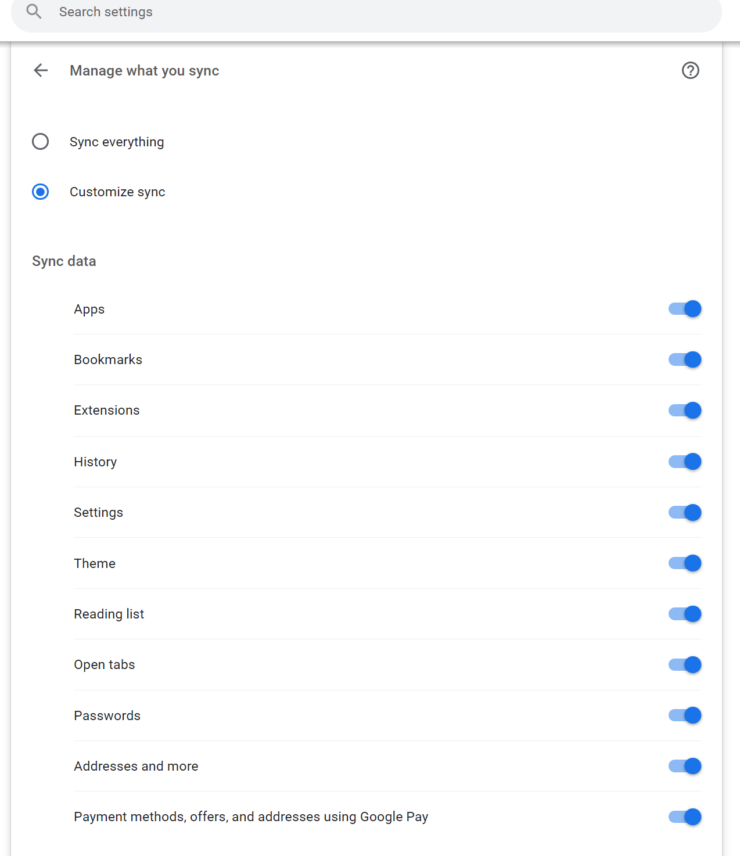The image depicts a web page with a search bar prominently displayed at the top. This search bar is grey with a magnifying glass icon on the left side, and the text "Search settings" is written in black within a dark grey bezel. Below this, the main page is white.

At the top of the main content, there is a black arrow icon pointing to the left accompanied by the text "Manage what you think" on the left-hand side. On the right-hand side of this line, there is a circular icon containing a question mark, likely intended for help or additional information.

Beneath this header, there are two round, clickable buttons. The first button, labeled "Sync everything," is not selected, while the second button, labeled "Customize sync," is selected.

Following this section, the text "Sync data" is displayed in bold black font. Below it, a list of terms is indented to the right, each accompanied by sliders. These sliders are pushed to the right, with a light blue background and a dark blue circle indicating they are enabled. The list of terms includes:

- Apps
- Bookmarks
- Extensions
- History
- Settings
- Theme
- Reading list
- Open tabs
- Passwords
- Addresses and more
- Payment methods
- Offers

Additionally, there is a term indicating "Addresses using Google Play."

The top bezel of the page is partially cut off on both the left and right sides, while the bottom portion of the page is also incomplete. The only indentation on the page is found within the list of terms.